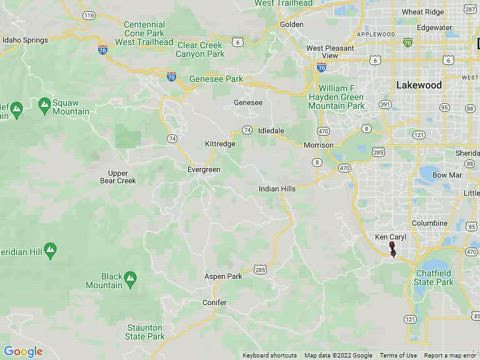This is a detailed description of a digital navigation map that is seen on a screen:

---

The navigation map displayed has several notable details and landmarks. At the bottom left corner, there's a label indicating "Google," while the bottom right corner contains references to "keyboard shortcuts, map data ©2013 Google, terms of use, report a map error." Surrounding these informational labels, the map itself is densely packed with various geographical and man-made features.

Prominently marked on the map is "Lakewood," along with other key locations such as "Shatfield State Park" and "Stockton State Park" towards the bottom right. Additional labeled regions include "Spadix, Black Mountain Riverside, Upper Berkeley, Evergreen, Indian Hills, Kiddridge, Ida-Del, Morrison," and "William F. Hayden Green Mountain Park." Several parks are also mentioned, such as "Gates Park, Clear Creek Canyon Park," and "Centennial Cone Park."

To the left side of the map, "Squaw Mountain" and "Meridian, Alabama" are visible, alongside "Black Mountain" and "Aspen Park." Conifer is situated towards the bottom. Within the map, a complex network of roads and interstates like 74, 78, 121, and 6 is visible, interspersed with numerous mountain roads depicted in white. Green patches represent forested or park areas, while gray patches indicate urban regions with buildings.

Additional towns and regions marked include "Edgewater, Bee Ridge, Arnold Springs," and "Columbine," located towards the bottom right of the map. At the top, the "West Trailhead" is highlighted in green. Overall, the map showcases a detailed mix of natural landscapes and urban developments, providing a comprehensive overview of the area.